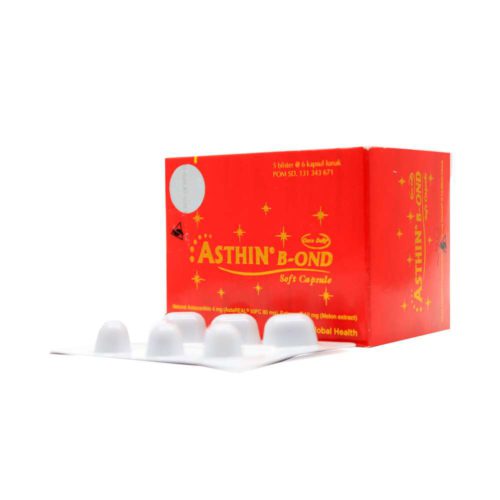The image depicts a red-orange box labeled "Ashton Bond" in gold text, with a small registered trademark symbol next to the brand name. Below the brand name, in smaller gold letters, it reads "soft capsule," accentuated by a streak of gold underneath. Surrounding the "Ashton Bond" text are numerous gold sparkles, adding a touch of flair. In the upper left-hand corner of the box is a white circle, potentially for a price tag, accompanied by a small black dot. The top right corner and the bottom edge of the box feature some indecipherable small text. Adjacent to the box is a solid white plastic bubble packet designed to hold the capsules, showing bulges where the capsules would fit if placed inside the box upside down. The entire setup is against a plain white background, with the box's orientation slightly favoring the left side of the frame.